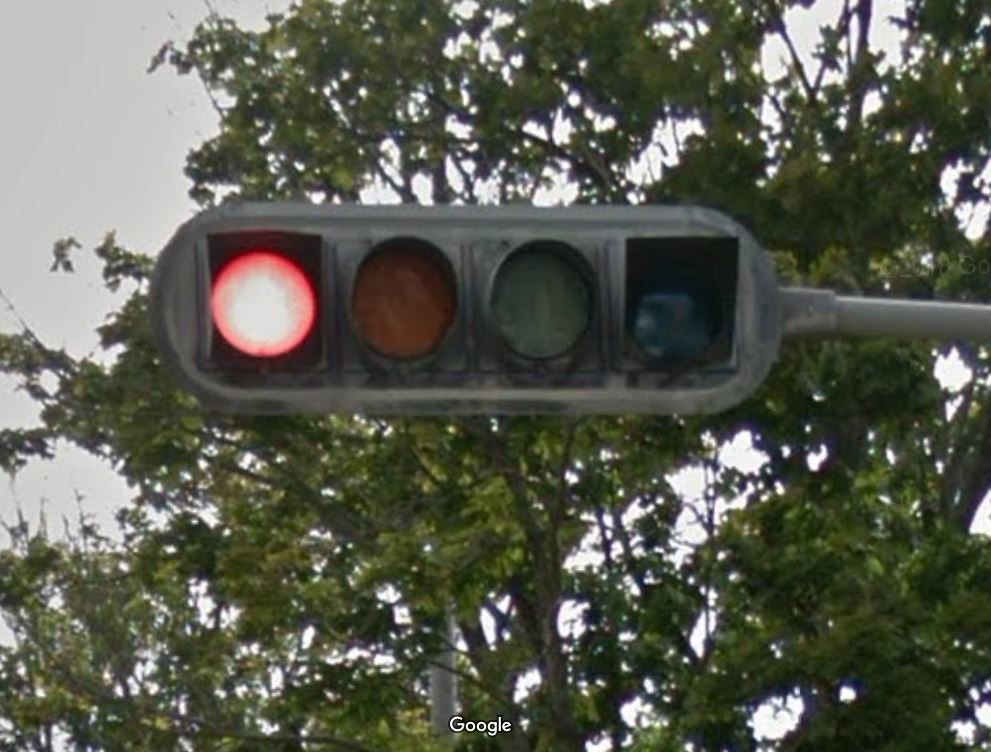The photograph captures an overhead traffic light suspended above a road, with a distinctive "Google" watermark in white text outlined in black at the bottom, indicating it is likely sourced from Google Street View. The image is closely cropped around the traffic light, which has a faded black casing and is attached to a silver pole extending off the screen to the right. The traffic light features four lamps: the leftmost lamp is a brightly illuminated red circle, signifying 'stop.' Next to it is an unlit yellow reflector, followed by an unlit green reflector, and finally, a slightly forward-tilting darker green lamp with a hood to shade it from sunlight, also unlit. The background reveals a dense array of dark green leaves and brown branches from surrounding trees, with sporadic patches of daylight creating a mix of darker gray and brighter white areas. The sky visible through the treetops appears overcast, adding to the soft, diffused lighting of the scene.